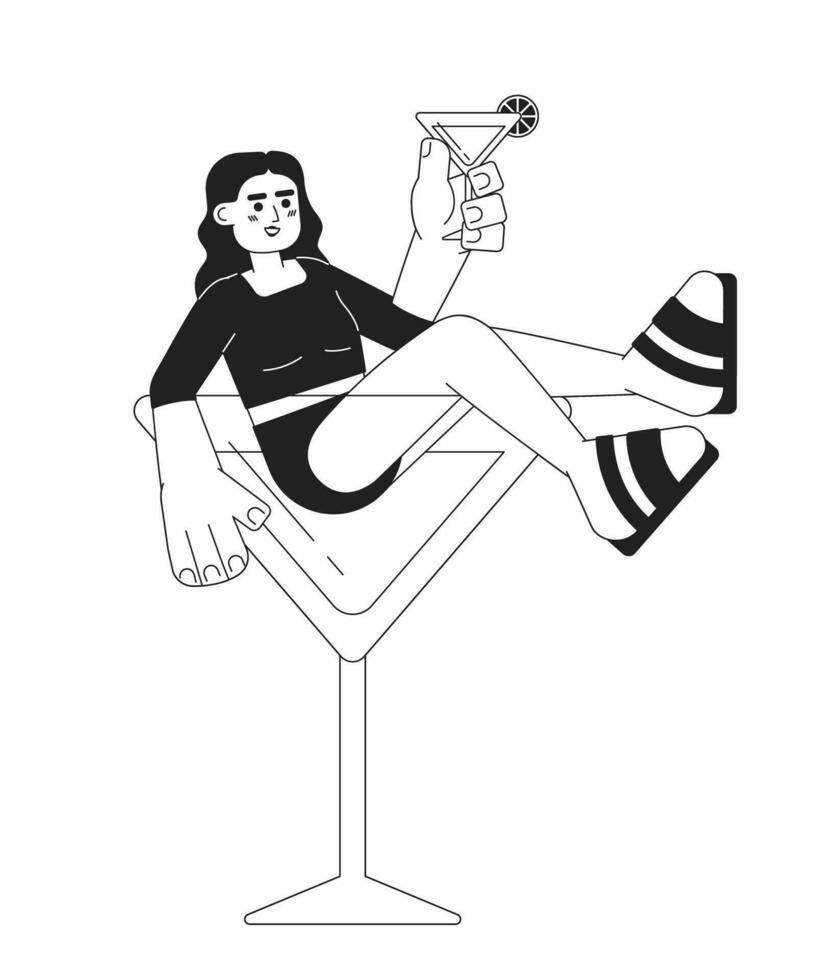In this black and white animated image, a woman is depicted in a simple, clipart-like style, sitting in a giant, thinly outlined triangular martini glass. Dressed in a black crop top with elbow-length sleeves, black bottoms akin to swimsuit bottoms, and black and white striped sandals, she is submerged up to her buttocks in the glass. The woman has exaggerated features: cartoonishly large hands and feet, and she holds another martini glass with a slice of citrus fruit on its rim in her left hand. Her facial features include long black hair, circular eyes, lines for eyebrows, and small lines on her cheeks suggesting blush. She has a slight smirk on her face. The image is presented in a portrait orientation with no background, emphasizing its stark, minimalist, and highly stylized aesthetic.